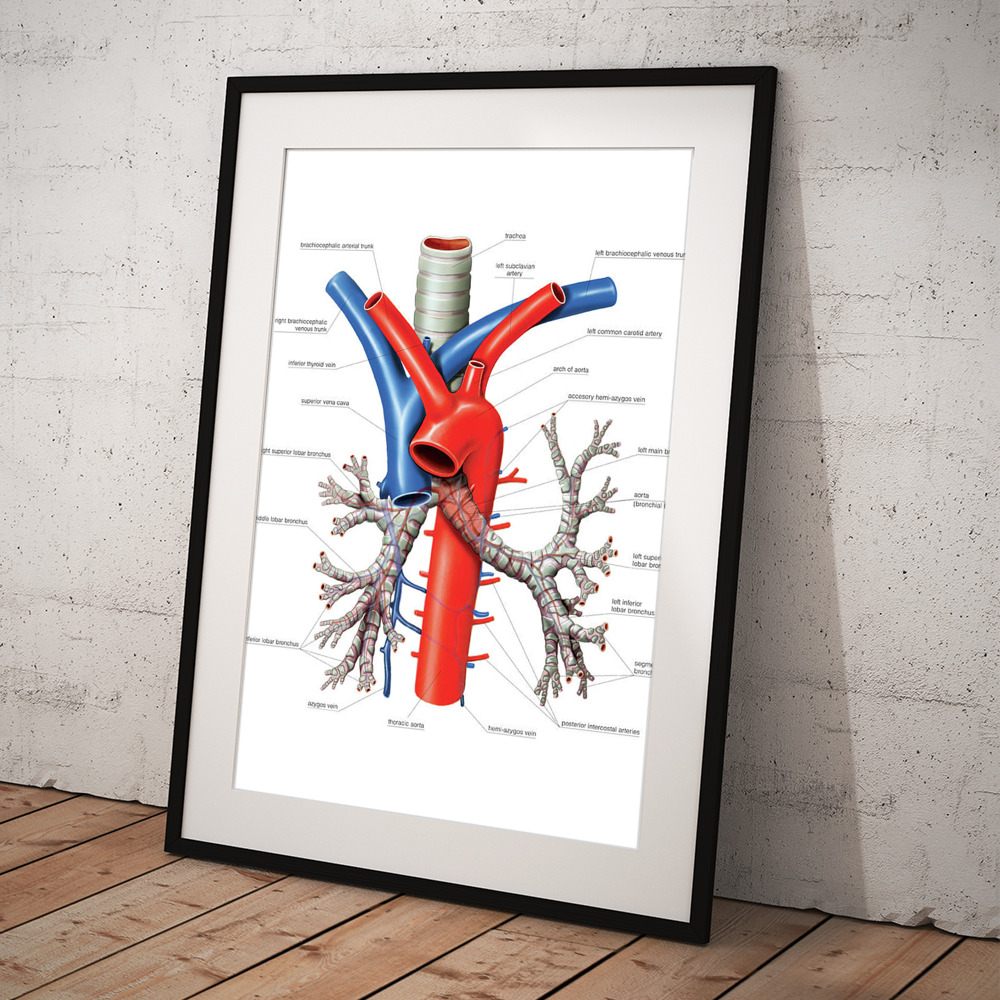This is a horizontal rectangular image of an anatomy diagram framed in black with a gray border. The poster itself is set against a white background and is propped on a wooden floor, leaning against a gray wall. The diagram features detailed illustrations of heart vessels without the heart itself, highlighting major arteries and veins. The central, prominent red artery, labeled as the left subclavian artery and left common carotid artery, extends in a candy cane-like shape with numerous branches at the top. Behind it, a blue Y-shaped vein, representing the venous system, extends downward. Both structures are connected to other systems, including the lungs. Noticeably, a silver circular tube labeled the trachea is positioned behind these vessels. The poster contains numerous small, detailed labels, including the arc of the aorta and the bronchus, making the intricate anatomical relationships clear despite the slightly angled view which may obscure some details.